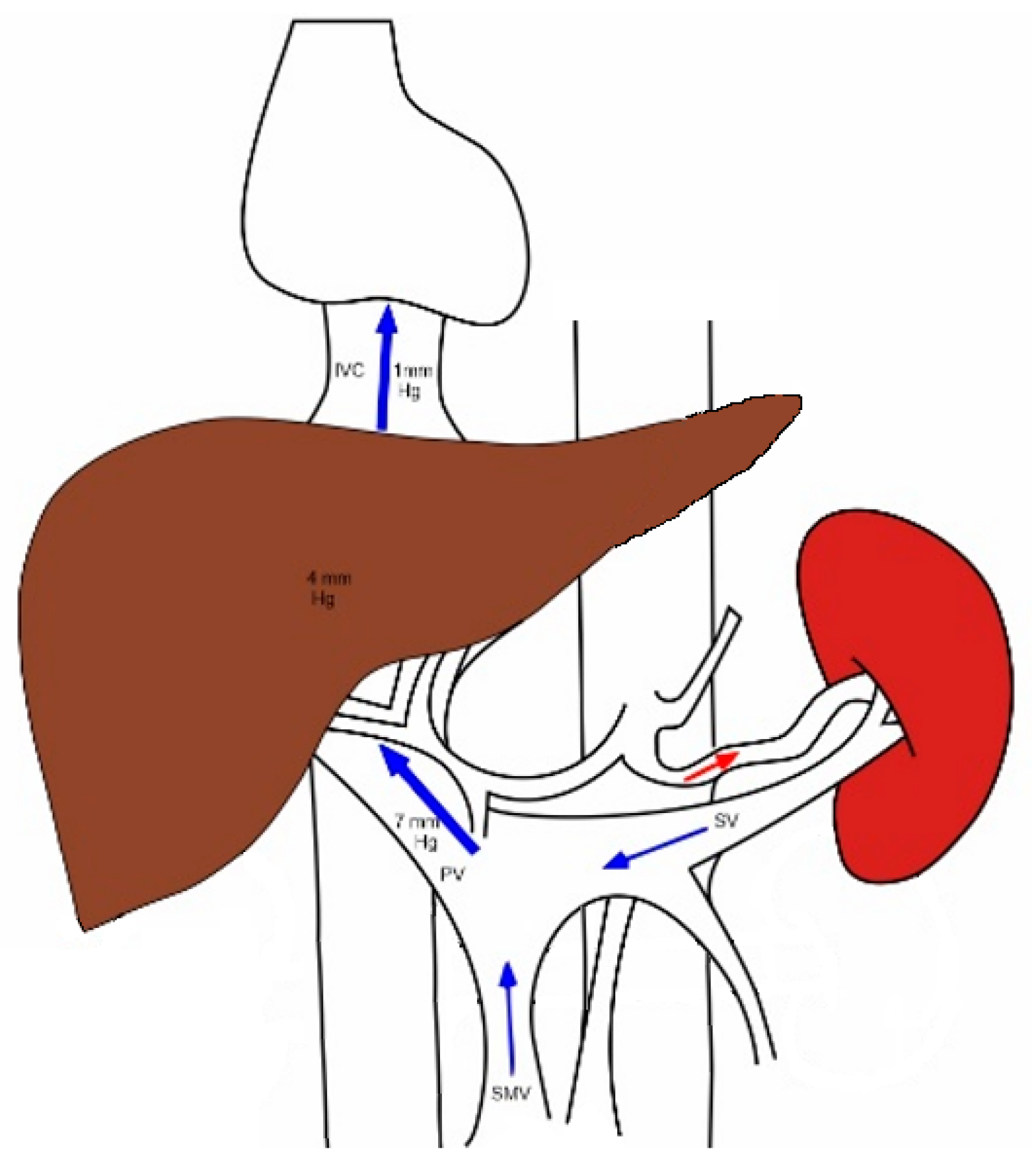This detailed anatomical drawing appears to depict blood flow between a liver and a kidney, both of which are distinctly filled in color amidst other outlined structures. On the left side of the diagram, a brown, rounded triangle shape likely represents the liver. Connecting to it are large, seemingly over-emphasized veins, labeled as SMV, SV, PV, and IVC. The IVC, in particular, is situated just above the liver, extending towards another unidentifiable, line-drawn organ that resembles a boot or cartoon foot, containing a blue arrow. This duct shows markings of "1 mm Hg."

On the right side of the image, there's a red kidney-shaped organ with a single red arrow pointing towards it, indicating blood flow from the liver. Blue arrows can also be seen leading from the kidney back to the liver. The drawing highlights blood pressure values, with "7 mm Hg" noted in one of the vessels and “4 mm Hg” marked directly on the liver. The overall crude rendering of the illustration, possibly completed using a basic computer program or pencil tool, presents an educational snapshot of abdominal anatomy focused on vascular pathways and blood pressure, albeit in a somewhat simplified and unclear manner.